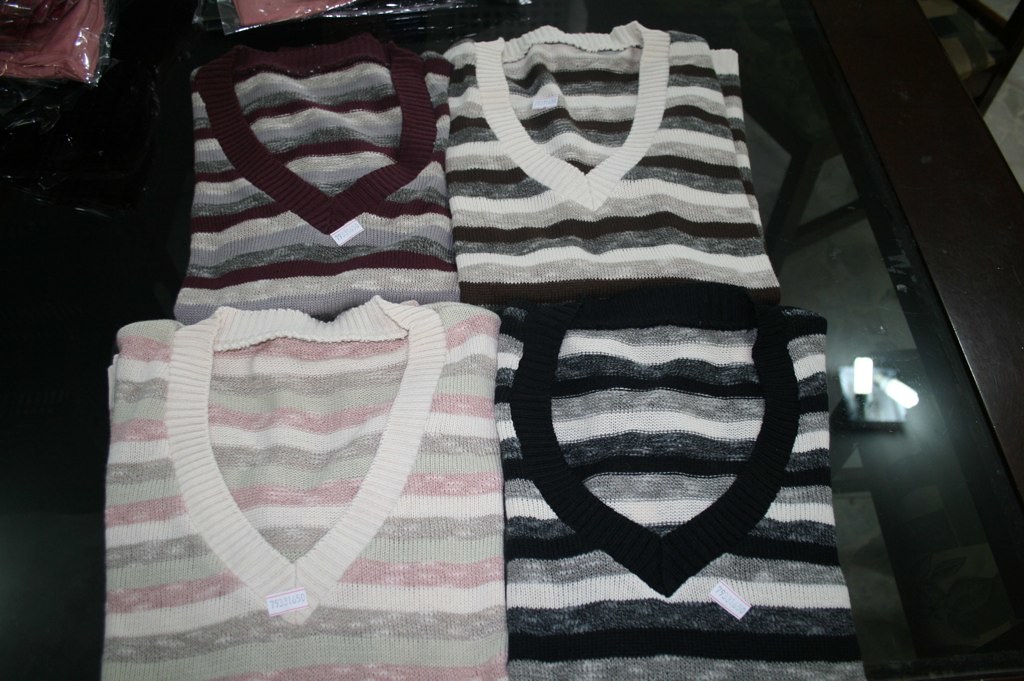This color photograph depicts a meticulously arranged display of four folded sweaters, side by side, with their contrasting ribbed v-neck collars facing up. The sweaters, each featuring distinct striped patterns in varying color palettes, are laid out on a sleek glass tabletop bordered by black. In the top left, a vibrant red shirt sealed in a plastic bag peeks into the frame, hinting at a store setting. The lineup includes a sweater with purple and pink stripes and a contrasting purple neck, a sweater with black and white stripes and a white neck, another with navy, white, and light blue stripes with a navy neck, and lastly, one with pink, brown, and white stripes complemented by a white neck. The sweaters are well-lit, with the light accentuating the glass table's reflectivity and revealing light gray flooring in the far background. The upper right corner shows the side of a black-framed dining room chair, further enhancing the scene's organized retail ambiance.